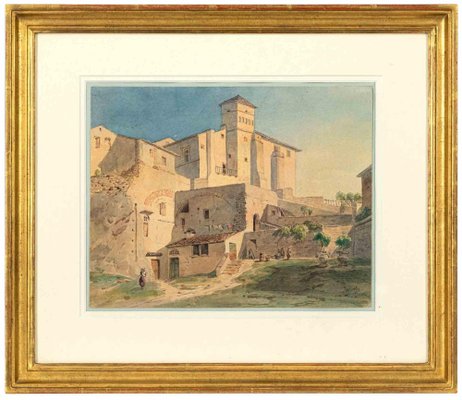This image depicts a framed painting that captures an idyllic Italian countryside scene, featuring what appears to be a large church or castle surrounded by smaller buildings. The painting is encased in an ornate gold frame, with a broad white or cream-colored mat board acting as a border between the frame and the artwork itself. Rendered in a watercolor style, the painting exudes a soft glow, with the lighting creating gentle shadows particularly evident in the foreground.

The buildings in the scene boast a mix of white, green, and beige tones, constructed from what seems like brown sandstone, with flat roofs and an overall rustic charm. The foreground is lush with green grass and bushes, where a solitary figure can be seen walking towards the prominent structure, emphasizing the grandeur and serenity of the locale. The bright blue sky and the warm, sunny atmosphere enhance the vividness and tranquil beauty of this Italian town, making the painting a captivating and detailed representation of an enchanting historical setting.